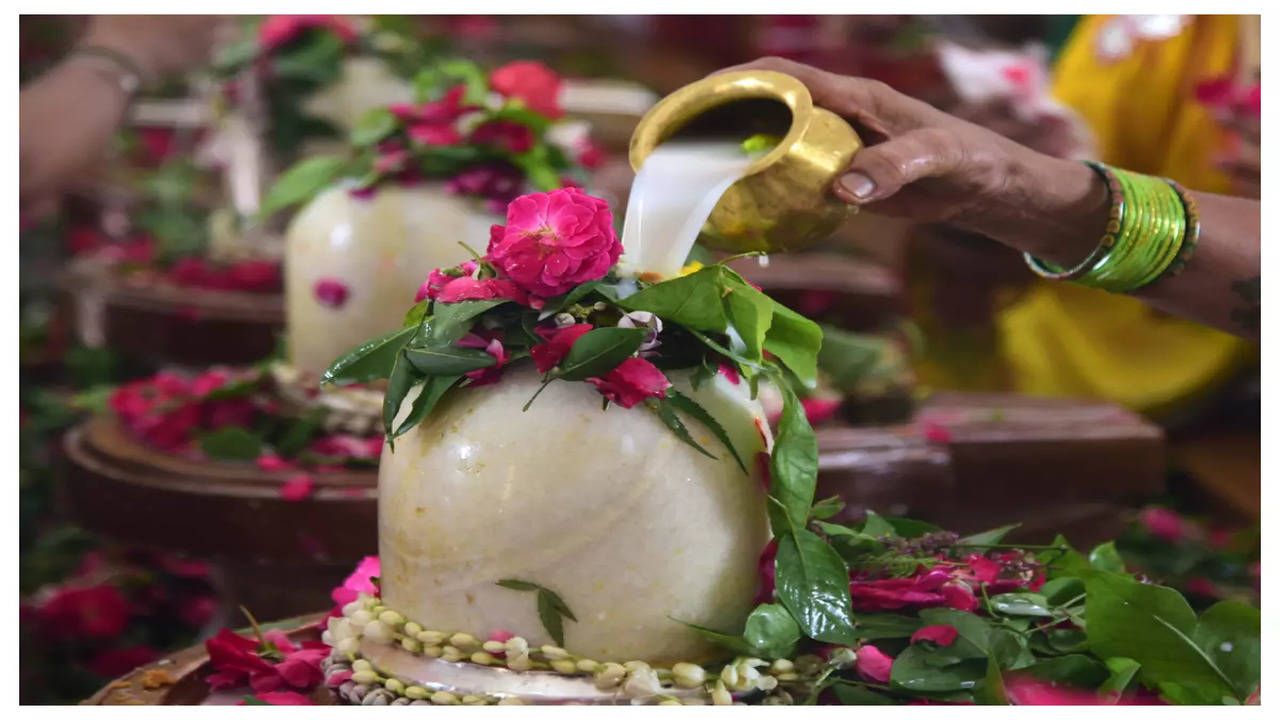The image features a scene with thick wooden tables arranged in rows, each adorned with a wide-bottomed, cream-colored ceramic vase narrowing to a small opening at the top. These vases, made of what looks like granite or marble, are filled with vibrant pink flowers and lush green leaves that drape gracefully over the sides. Surrounding the base of each vase are earthy green beads. In the foreground, a light tan arm extends into the frame from the right, adorned with a bead bracelet. This person is pouring a white, milky liquid from a small, gold cauldron into one of the vases, which sits on a rust-colored tin dish. The background shows a continuation of the floral arrangements and vases on similar wooden tables.